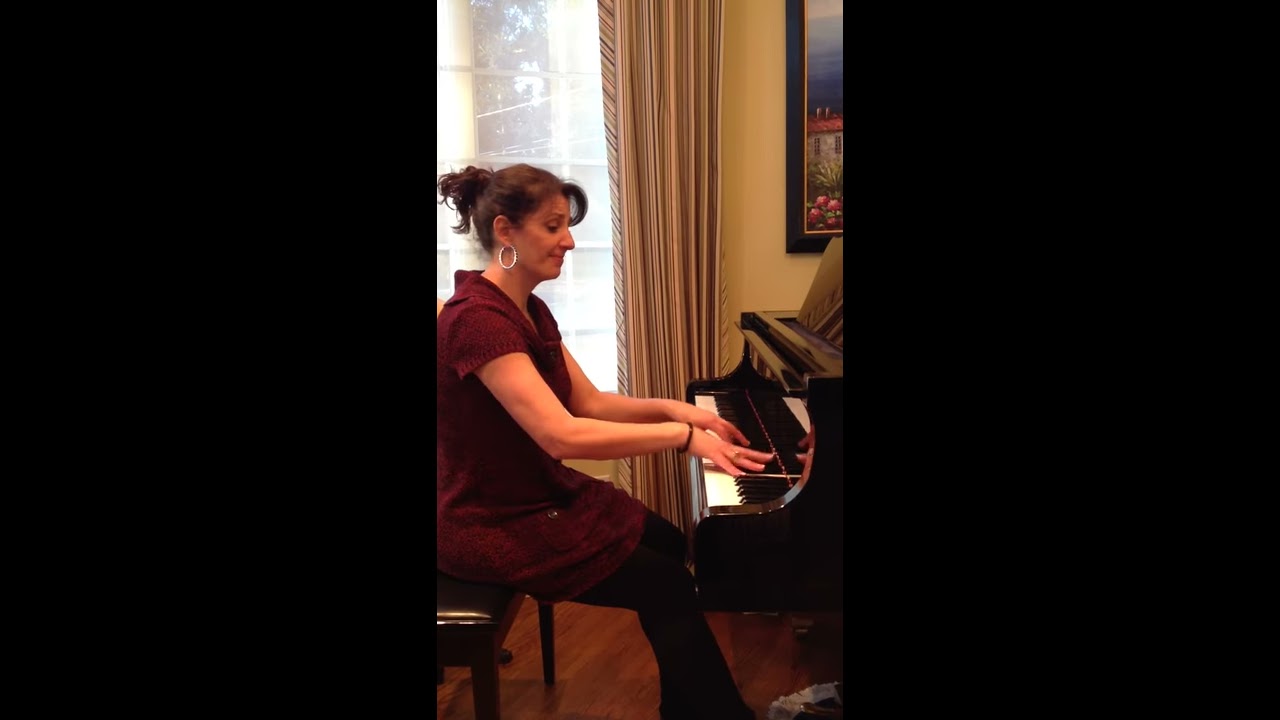This image, presented in a portrait orientation against black landscape borders, captures a middle-aged woman enthusiastically playing a wood brown piano in what appears to be a living room. The woman, with her dark hair pulled back into a ponytail, is dressed in a textured, short-sleeved, reddish-burgundy dress paired with black tights. She is adorned with large silver hoop earrings and a black bracelet on her right wrist. Seated on a piano bench, she focuses intently on the piano keys while a soft smile graces her face. The background features a painting partially visible to the right, a yellowish wall, beige curtains, and a window through which daylight streams, casting a warm glow across the scene. The wooden floor beneath her and the overall photographic realism bring further depth to the composition.